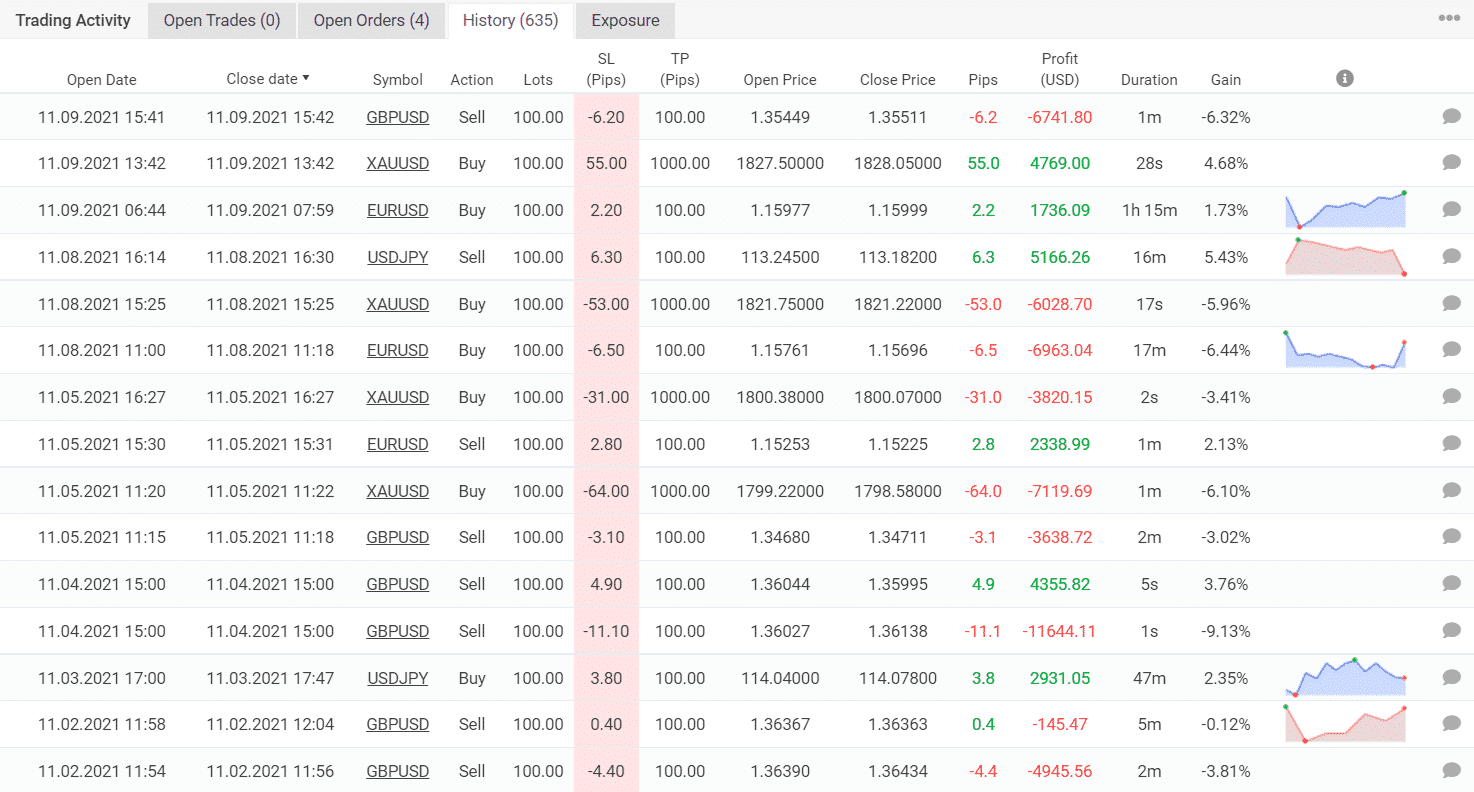This screenshot, captured from an unspecified trading website, prominently features two navigation menus at the top. The first menu comprises options such as: Trading Activity, Open Trades, Open Orders, History, 635, and Exposure. Directly beneath, a secondary menu bar lists several columns titled: Open Date, Closed Date, Symbol, Action, Lots, SL Pips, TP Pips, Open Price, Closed Price, Pips, Profit USD, Duration, and Gain. 

The columns are populated with various dates, numerical values, and stock symbols, detailing the intricate activities and outcomes of different trades. Notably, some columns towards the end display blue or pink graphs, although these graphical representations are not present in every entry. 

An outlined column in pink, labeled SL Pips, catches attention with its array of numerical values indicating stop-loss pips, ranging from -64 to 490, demonstrating a fluctuating trend. The specific values listed are: -6.2, 55, 2.2, 6.3, -53, -6.5, -31, 2.8, 64, -64, -3.10, 490, 4.90, -11.1, 3.8, 0.4, and -4.4.

This detailed screenshot encapsulates the extensive and meticulous data essential for evaluating trading performance, with a specific focus on the stop-loss pips column.